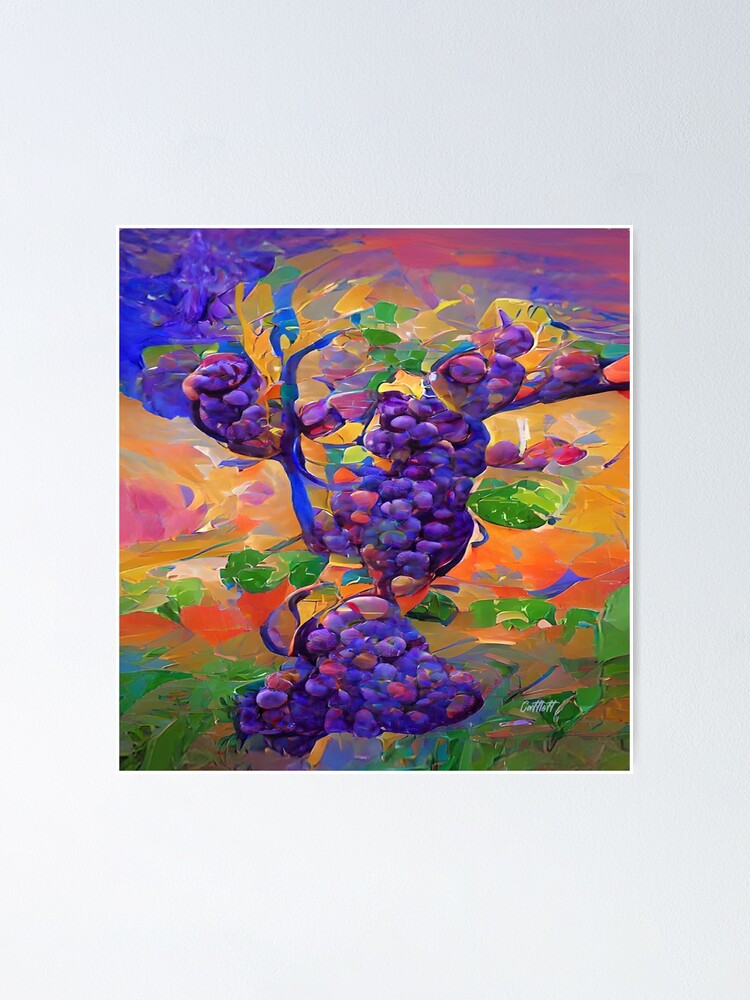The image is a vibrant and abstract painting of a grape vine featuring three prominent bunches of ripe, purple grapes. The canvas is enclosed in a very thin white frame and is mounted against a grayish off-white background. The art piece employs broad brush strokes and swirls, heavily influenced by Impressionist design, giving the painting a textured and dynamic appearance. The grapes are surrounded by a colorful array of hues, including reds, blues, yellows, dark greens, light greens, and oranges. These colors create an impression of leaves, grass, and a sky that blended together in a surreal landscape. The background showcases an orangey-yellow horizon, possibly depicting a sunset or sunrise, which adds a trippy, dreamlike quality to the overall image. The artist's signature, "COTTSTT," is located in the bottom right-hand corner of the painting.